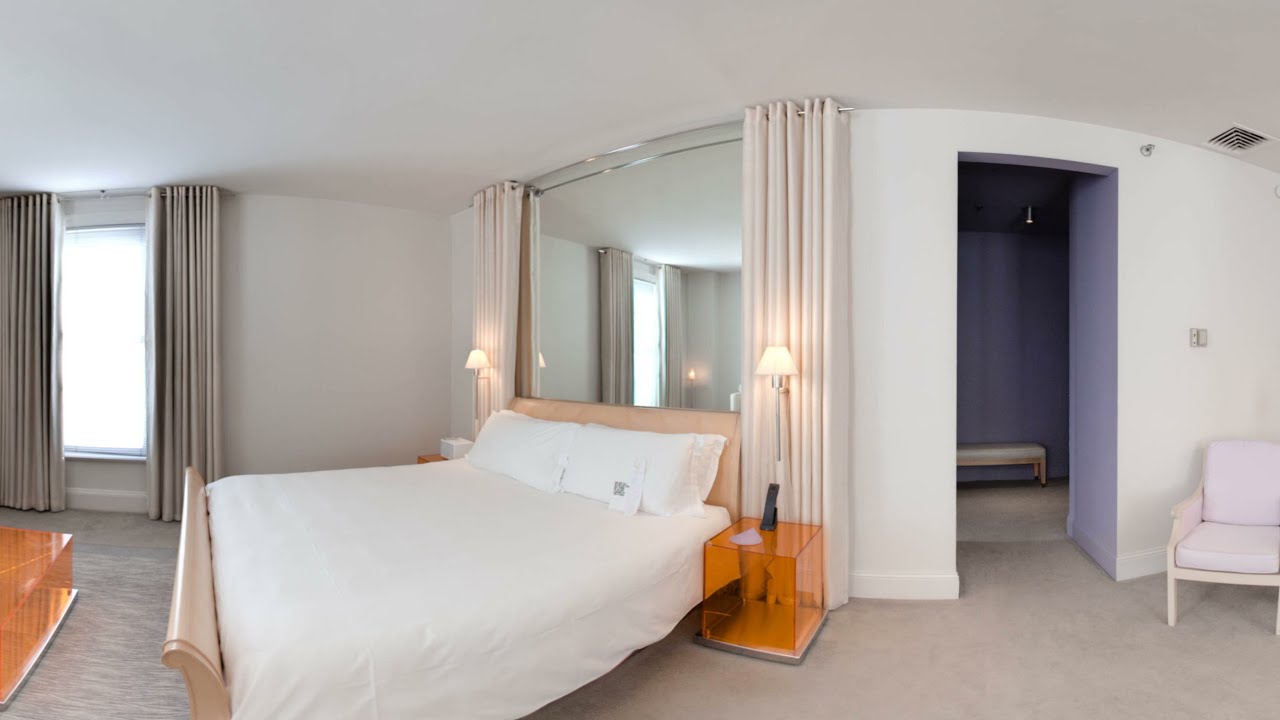This image depicts the interior of a modern and spacious hotel bedroom. Dominating the left side of the room, a large bed dressed entirely in white with a sleek white blanket and two king-sized pillows takes center stage. Above the headboard—a modern fixture matched with a sleek baseboard—is a floor-to-ceiling mirror framed by tan curtains. On either side of the bed, square nightstands hold sculptural orange plastic lamps, contributing to the post-modern aesthetic that includes other pieces like an odd, ultra-modern ottoman in the left-hand bottom corner. Adjacent to the bed on the left, there's a window adorned with taupe curtains partly open to reveal beige-taupe carpeting. To the right, the room features a doorway, beyond which a small, white-upholstered chair and a bench are visible, suggesting this could be an entrance to an attached bathroom. The overall decor is generic yet stylish, with defining touches of modernity and simplicity that would appeal to a hotel guest looking for mid-tier luxury.